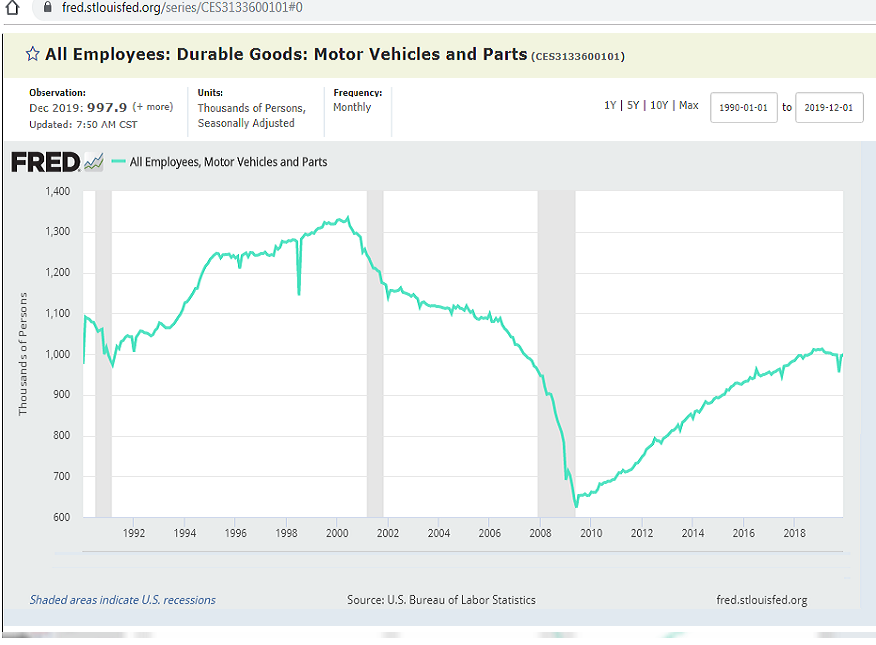The image features a detailed chart prominently centered, depicting a line graph titled "All Employees, Durable Goods, Motor Vehicles, and Parts." The line, colored in green and fairly jagged, represents the number of employees in these sectors from 1992 to 2018. The x-axis marks the years, and the y-axis appears to denote the units, perhaps in thousands of persons. Above the graph, there are detailed headings and descriptors outlining the units, frequency, and observations, while below the chart, the source is attributed to the US Bureau of Labor Statistics. The background of the chart is grey, with the label "FRED" appearing in bold, black capital letters.